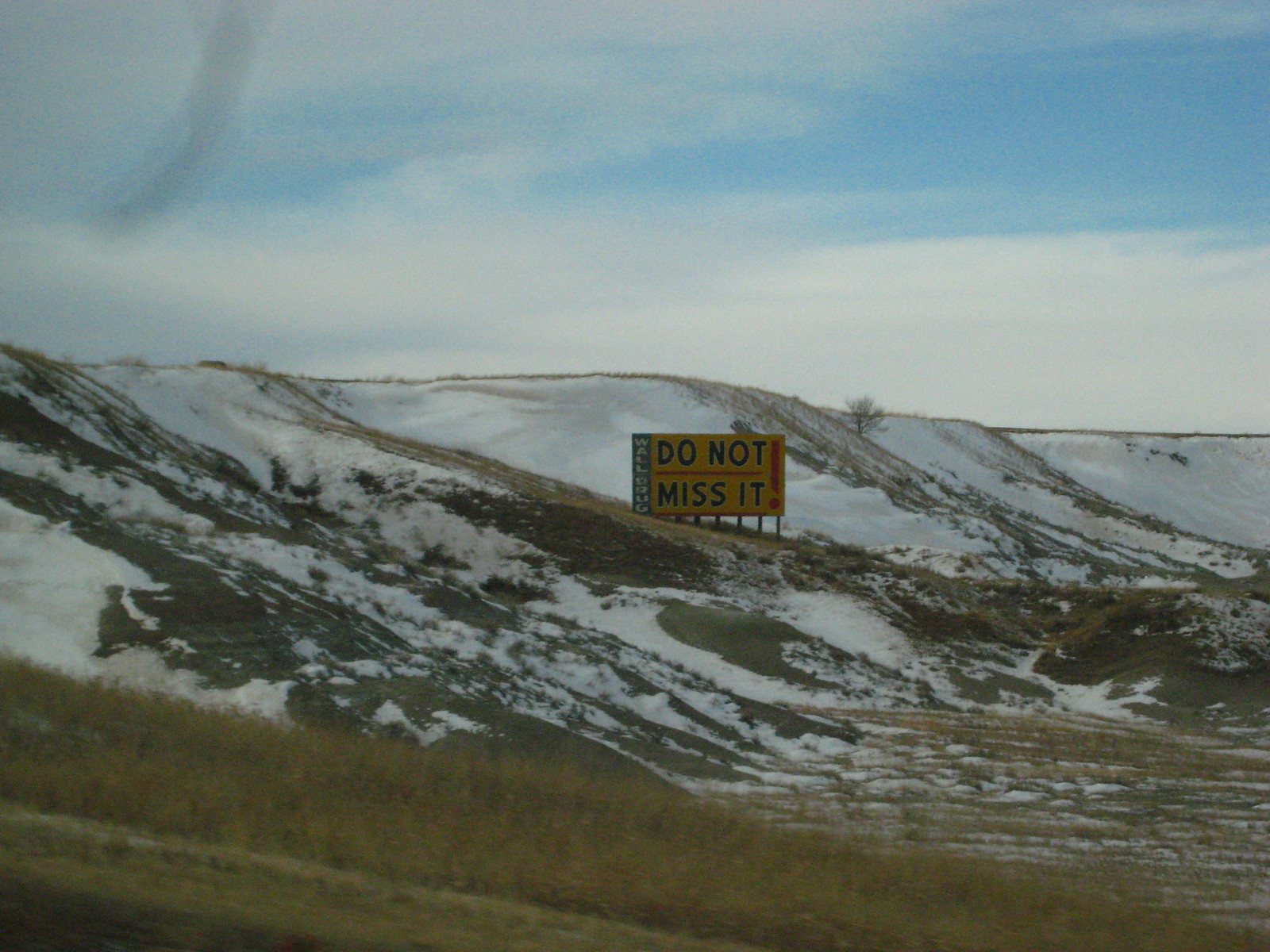The image shows a bright, daytime scene with clear blue skies hosting a few loose, fluffy clouds. The foreground on the bottom left features a field with dull green and brownish grass, indicative of a rugged, possibly winter-ravaged landscape. The middle ground reveals a series of grayish-brown hills peppered with patches of melting snow, exposing the brown soil and sparse vegetation beneath. Centrally positioned on one of these gently sloping hills is a striking rectangular sign. Set upon sturdy wooden posts, the sign has a vibrant yellow background and bears a prominent message in bold black capital letters: "DO NOT MISS THIS." The phrase is divided by a horizontal red line, and an emphatic red exclamation mark punctuates the statement. Although some distant trees can be faintly seen, the landscape seems largely desolate, exuding a sense of raw, untouched nature.